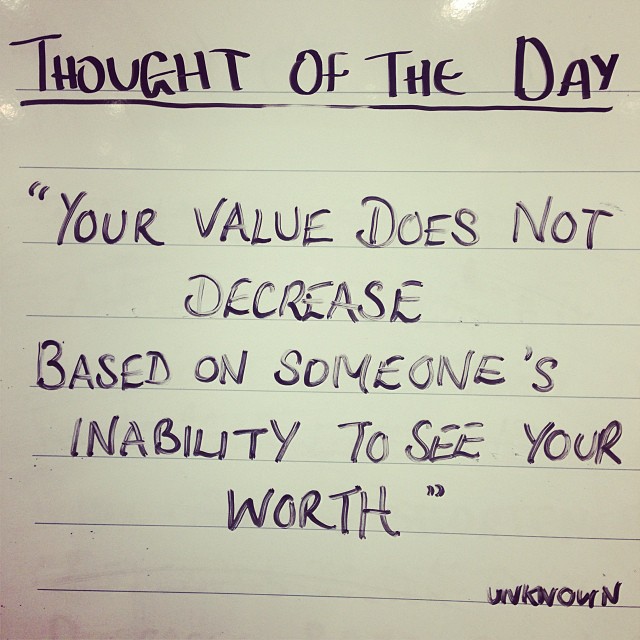The square-shaped image features a piece of white lined paper with a handwritten inspirational quote. At the top, in bold black Sharpie text, is the underlined heading "Thought of the Day." Beneath this, written in black ink and enclosed in quotation marks, is the motivational message: "Your value does not decrease based on someone's inability to see your worth." The words show slight fading, suggesting the pen was running low on ink. In the bottom right corner, the author is denoted as "Unknown." The paper appears to be photographed with light coming from the upper right, causing some slight tilting of the lines to the right. The entire quote is written in regular, non-cursive script, reminiscent of grade school lettering.